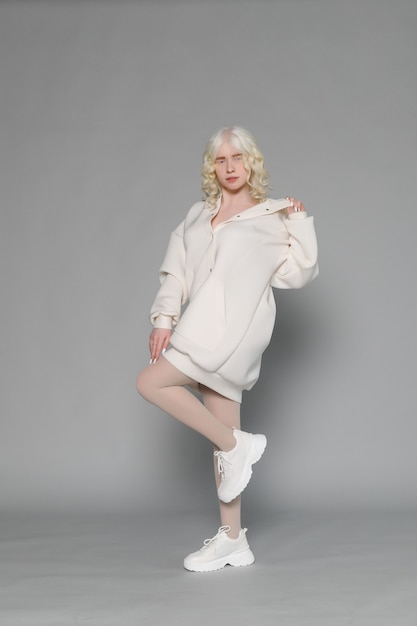The photograph is a full-color, vertically rectangular, staged modeling shot taken indoors under artificial lighting. The background consists of a seamless gray wall and floor with no borders or writing. The focus is a very pale, platinum blonde-haired Caucasian female with pronounced brown eyebrows and uniquely expressive eyes. She wears all-white attire: an oversized white sweatshirt that extends to her thighs, white tennis shoes, white nylons, and white fingernails. Her hair is straight at the top, transitioning to curls at the shoulders. Striking a dynamic pose, her right leg is curled up with the knee bent and the foot touching her left knee. She gazes directly at the camera, her body slightly twisted, contributing to the stylish, almost surreal atmosphere of the shot. The clean and coordinated fashion statement, accentuated by the monochromatic white outfit against the minimalist gray background, suggests this is a professional modeling image.